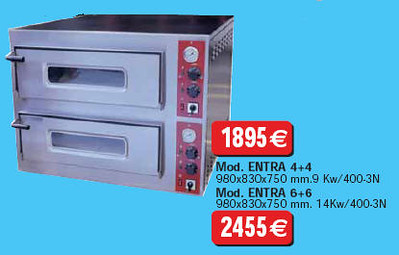The image depicts a landscape-style advertisement for a sleek, double-stacked dual toaster oven. The toaster oven features a shiny, metallic silver casing composed of metal or steel. Each of the two oven compartments includes a clear glass window and black handles for easy access. The right side of the appliance is adorned with red panels housing black-colored buttons and controls, including temperature settings, two knurled knobs, and several switches.

Prominent in the image are two price tags: one for 18.95 euros and another for 24.55 euros. Accompanying these price tags are technical specifications: for the first model, 'mod Entra 4 plus 4', with dimensions of 980 x 830 x 750 millimeters and a power rating of 9 KW/400-3N; for the second model, 'mod Entra 6 plus 6', with the same dimensions but a power rating of 14 KW/400-3N. The background of the advertisement is a vibrant teal light blue, which accentuates the modern and appealing design of the toaster oven. This graphic appears to be professionally designed, with text in a foreign language emphasizing the advanced features and efficiency of the appliance.